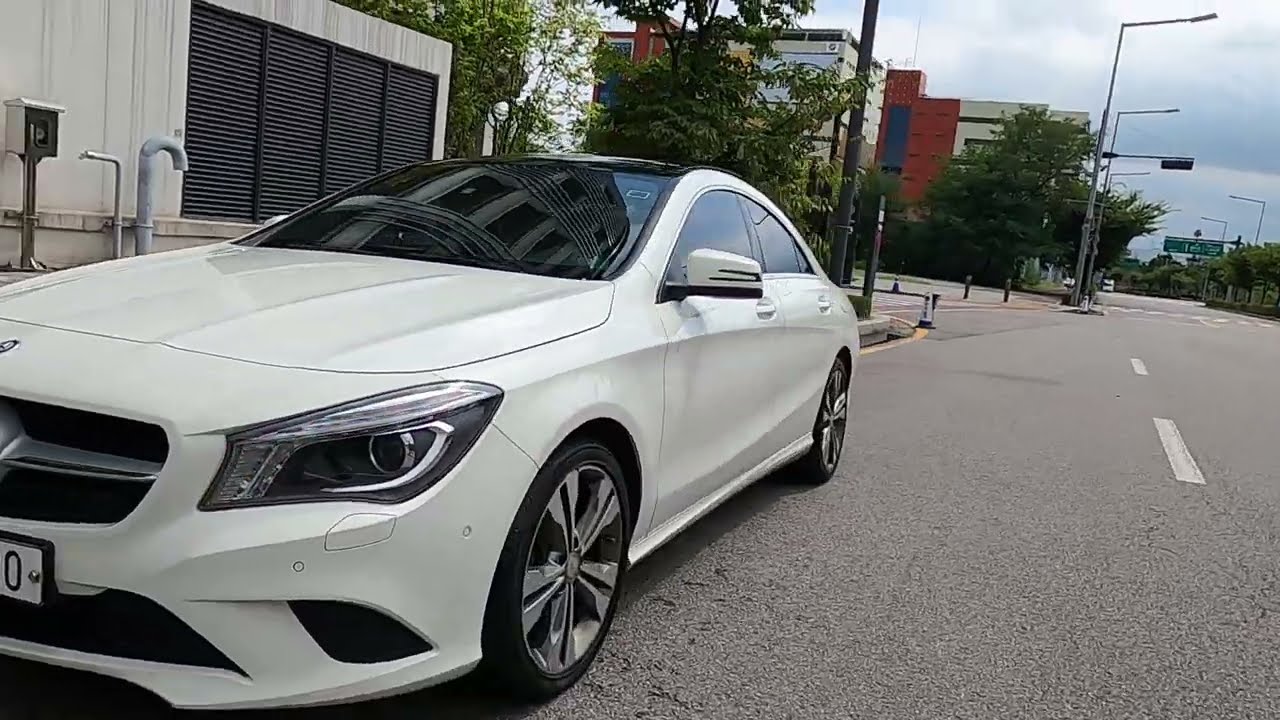In this image, we observe a typical white sedan parked in the bottom left corner of a roadway scene. The road runs along the right side of the image and features various markings and lights indicative of a small city's street. The scene is captured during the middle of a cloudy, dry day, adding a subdued lighting to the environment. 

A few buildings are positioned mainly in the top and top right segments of the image, lending an urban backdrop to the scene. Additionally, behind the car, there is a garage with a folded door, reminiscent of those found at rail or bus stations. Just past the car, street poles and trees add depth to the backdrop, with no text present anywhere in the image. The overall palette includes off-white, gray, black, white, red, green, and light blue colors, reflecting the muted tones of a typical small city setting.